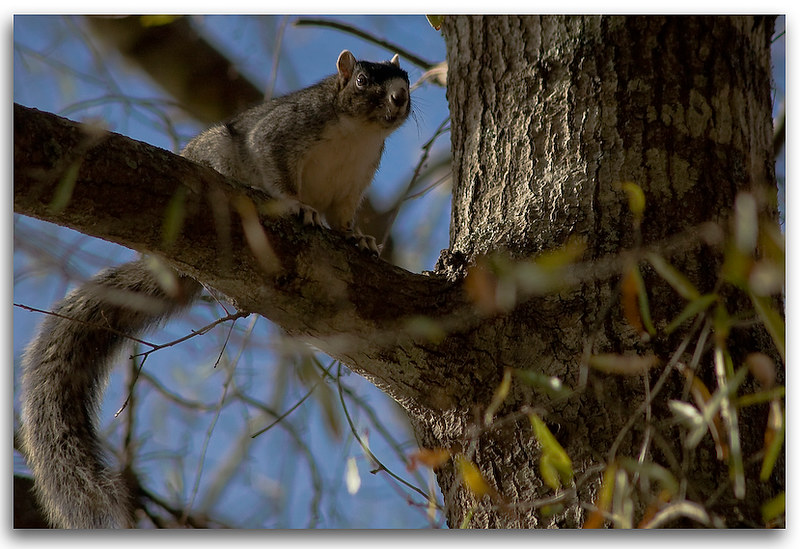This captivating close-up image features a plump squirrel perched on a branch extending from the left-center towards the left of the frame. The tree trunk occupies the entire right half of the image, showcasing its textured bark. The squirrel, with its dark eyes, black nose, and prominent whiskers, gazes almost directly at the camera, adding a sense of curiosity and engagement. Its front paws firmly grasp the top of the branch, with a notably long and fuzzy gray tail that curves down towards the bottom left corner. The background reveals a bright blue sky dotted with blurry branches and small, possibly shedding leaves, which might indicate either the season or the tree's variety. Sunlight filters through, highlighting the squirrel's fur, which transitions from gray to light gray-white towards its rear. The entire scene is bathed in natural daylight, emphasizing the wild and serene environment in which this endearing creature resides.